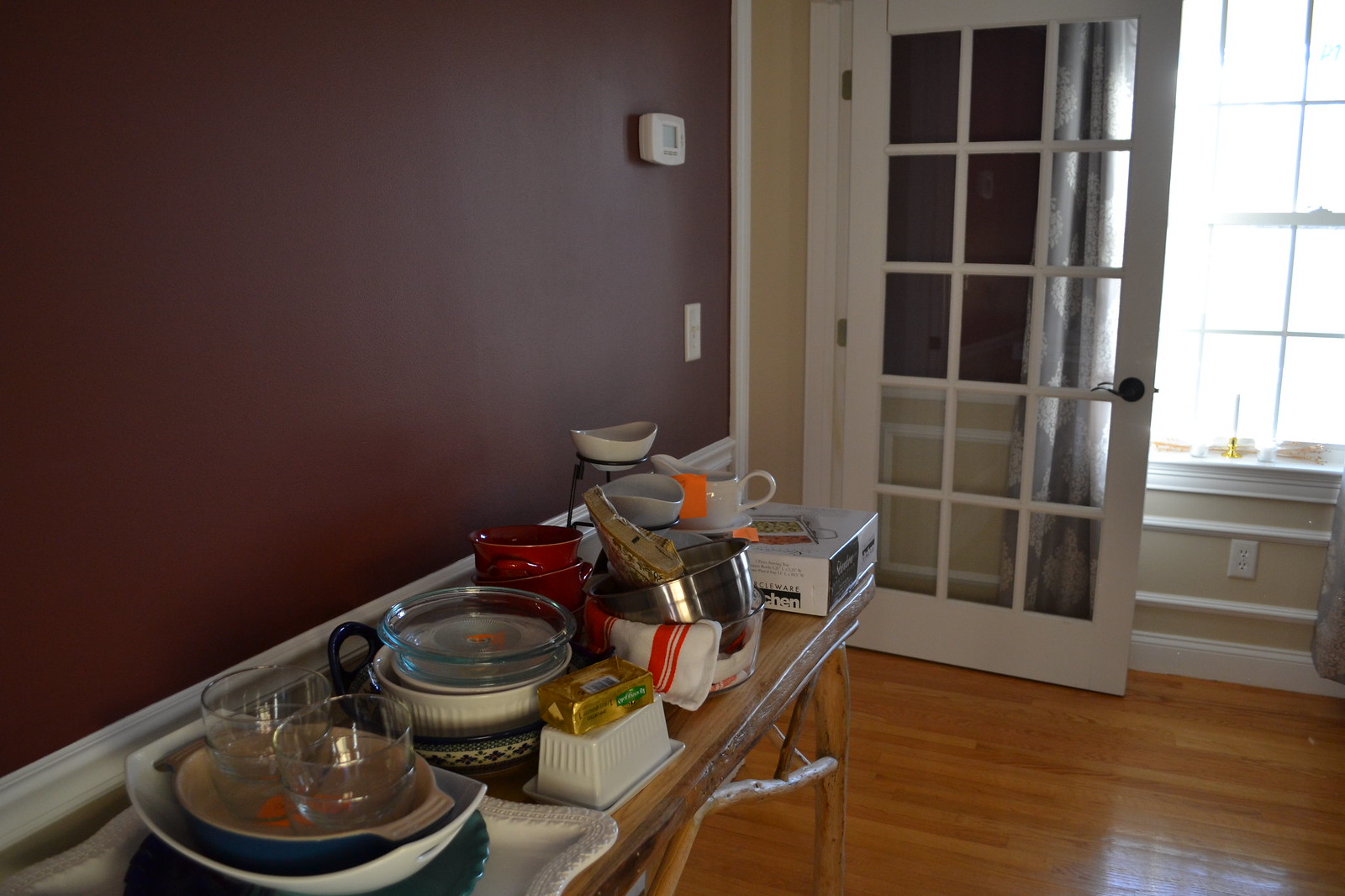The image depicts a room with gleaming hardwood floors. The dominant feature of the room is the back wall, which is painted maroon and adorned with a white thermostat and a switch. This wall also has a white door that is partially open, revealing 15 small glass windows arranged in a grid pattern of three rows of five.

The right side of the back wall is primarily white with elegant white trim, capturing an abundance of sunlight streaming through a large window. This creates a bright and inviting atmosphere.

A long, skinny table runs along the maroon section of the wall, displaying an array of decorative fish. Adjacent to this, a tall ladder leans against the wall, contributing to the room's eclectic decor.

On the side wall, there is a traditional round table made of real wood, featuring intricate branch-like carvings. The table is tastefully set with various items: a white porcelain platter, blue round candy dishes, clear cups, grainy woven mats, and neatly folded towels, accented by a leather accessory.

The room exudes a sophisticated yet cozy ambiance, balancing rich colors and natural light with carefully selected decorative elements.